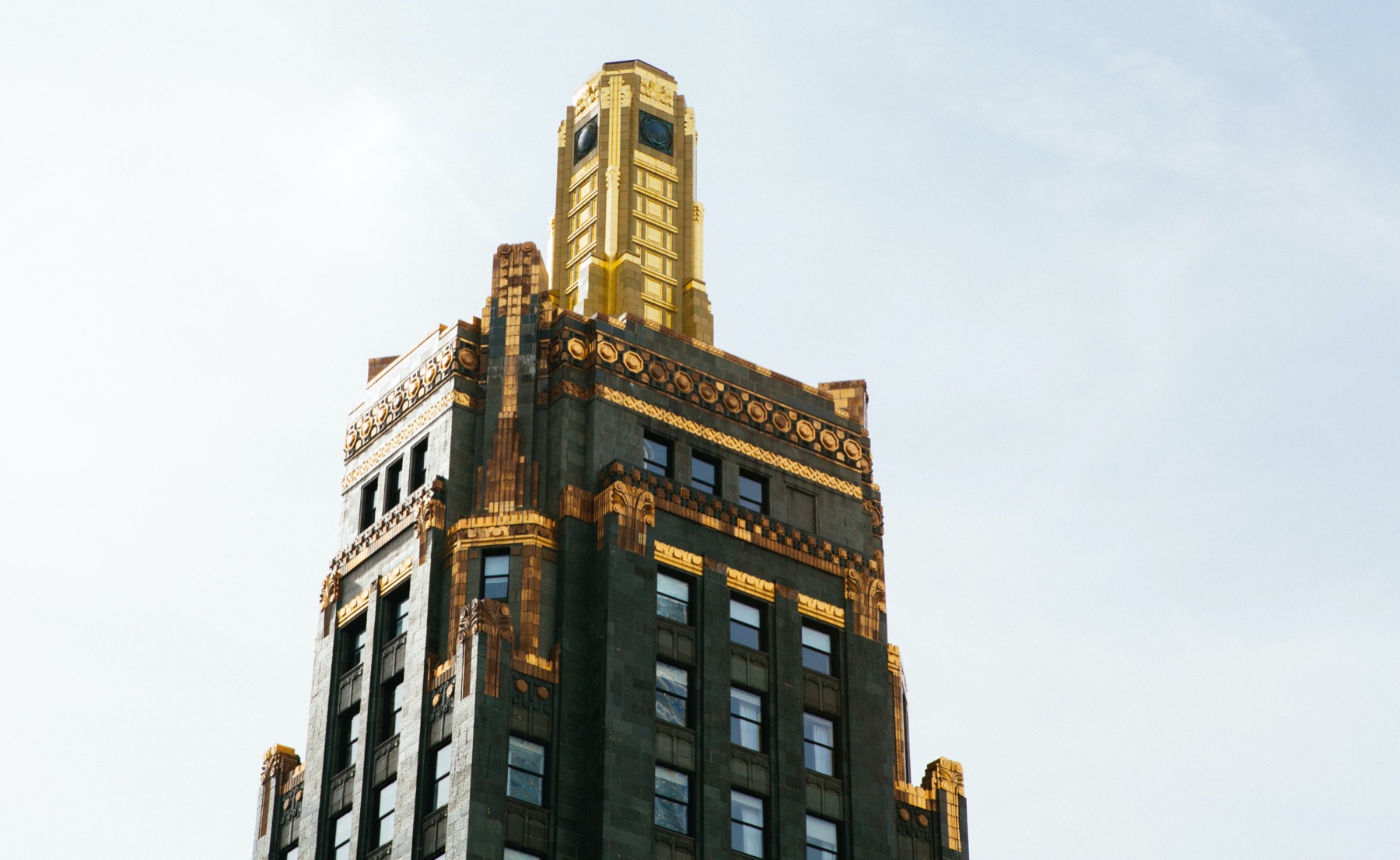The image depicts a high-rise, possibly Art Deco-style skyscraper rendered in a striking combination of black and gold. The photograph captures the upper portion of the building against a backdrop of a partly cloudy blue sky, suggesting a bright sunny day. The building itself is predominantly black, adorned with elaborate gold accents. The very top features a gold, ornate tower-like structure embellished with intricate details and surrounded by black, window-like elements with a bubbly texture. Below this, the roof and upper floors showcase a series of windows tinted with a hint of blue, flanked by gold trims and designs—including gold lines, circles, squares, and ram-shaped motifs—distributed gracefully across the structure's facade. The overall aesthetic hints at a historic elegance reminiscent of the 1930s or 40s, merging modern grandeur with classic architectural flair.